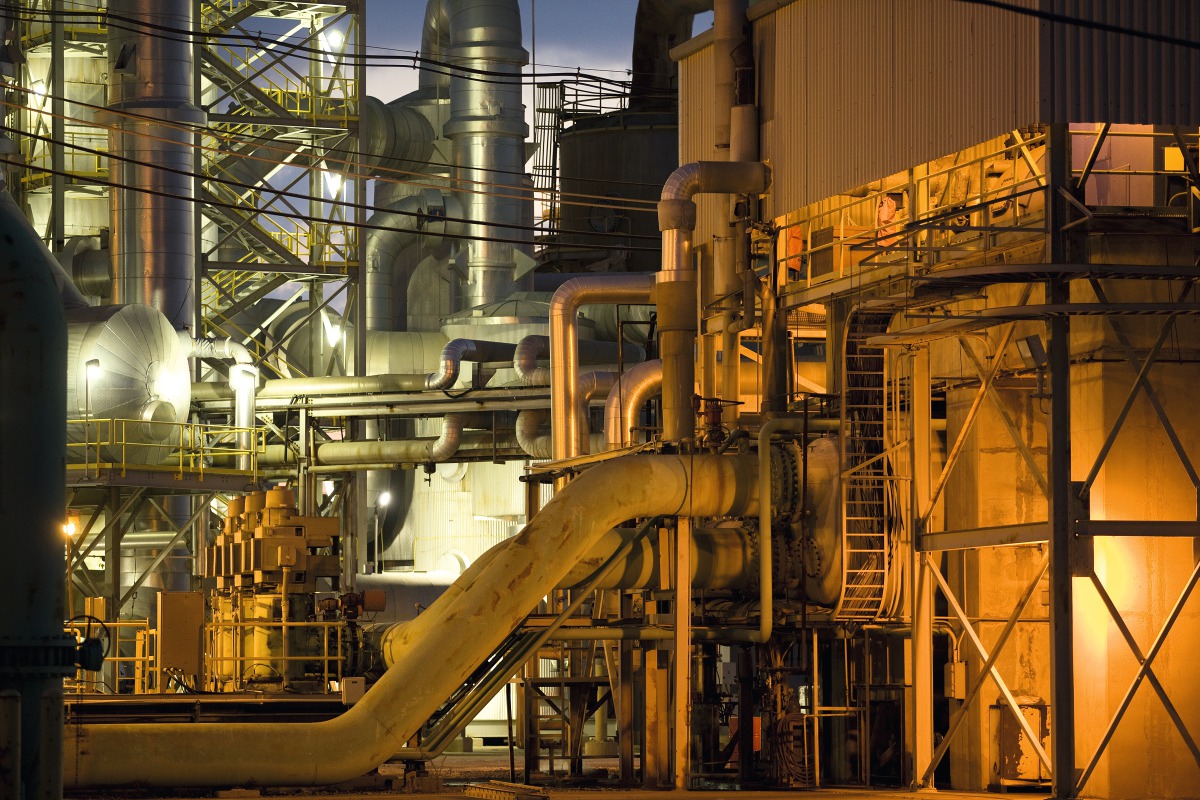The image showcases a side view of an industrial power plant or factory, marked by a plethora of metal tubes and railings that give it a strikingly mechanical and intricate appearance. An orange light in the bottom right corner illuminates parts of the building, casting a warm glow over the metal structures and highlighting details in the environment. Amidst these components, ladders and staircases are visible, adding to the complex and potentially hazardous atmosphere. The background features the sky, a dim blue color indicating the time around sunset or dawn, creating a serene juxtaposition to the bustling industrial scene. The image is clear and well-lit, capturing the essence of a dynamic and meticulously constructed industrial landscape.